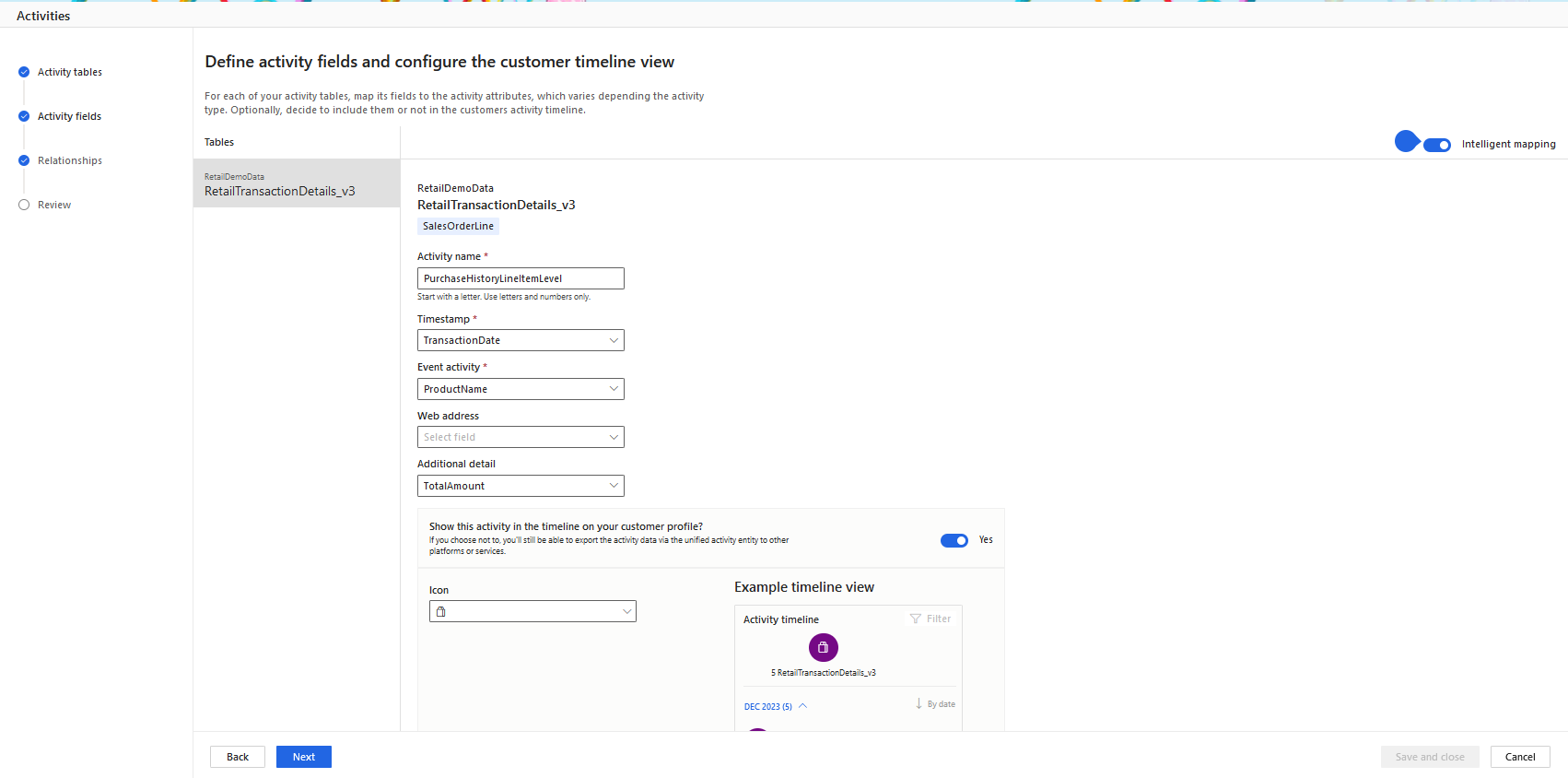This screenshot captures a detailed view of a website interface, likely viewed on a laptop or desktop computer due to its horizontal orientation and screen size. The website appears to be a form or setup process, specifically for configuring activity fields and customer timelines. The interface displays a section titled "Activities," featuring options for defining activity fields and mapping them to activity attributes. Users are prompted with instructions such as "for each of your activity tables, map the fields to the activity attributes, which vary depending on the activity type." 

Several fields are available for input, including Activity Name, Timestamp, Event Activity, Web Address, and Additional Details. A decision diagram is present, allowing users to choose whether to display each activity on the customer profile, with selectable "Yes" or "No" options. At the bottom of the page, control buttons offer functionalities including "Save and Close," "Cancel," and a "Next" button to proceed to the following step. Additionally, a toggle button for "Intelligent Mapping" is activated, suggesting some level of automated assistance in the mapping process. This comprehensive user interface aids in the meticulous configuration of customer activity tracking.